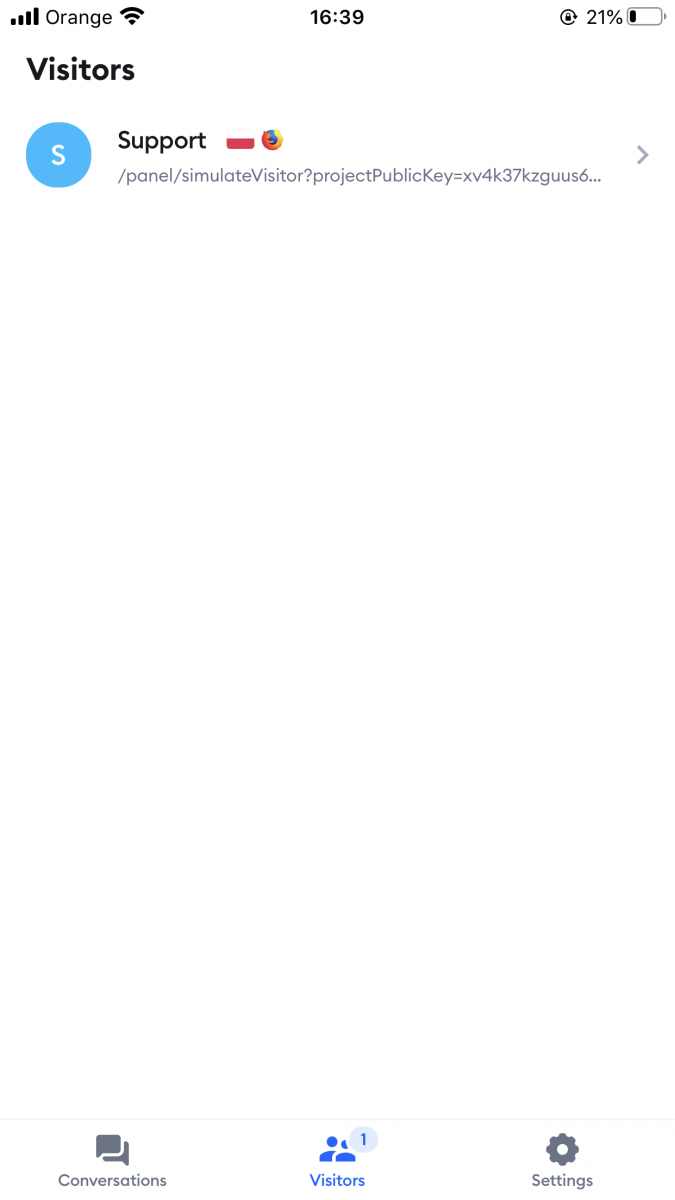The web application interface presents a comprehensive and structured layout. At the bottom of the page, three distinct tabs are available: Conversations, Visitors, and Settings. The "Visitors" tab is highlighted in blue, featuring a small notification circle with the number one, indicating there is one active visitor. 

The top of the page displays several status indicators including the signal strength, the connected network labeled as "Orange," a Wi-Fi strength indicator, the current time (16:39), and an additional icon resembling a small letter enclosed in a circle, whose function is not immediately clear. It also shows the battery's charge level, which is at 21%, with the battery icon visually confirming the low charge.

Dominating the main section of the screen, bold black text spells out "Visitors" in sentence case, situated in the upper left portion just below the signal strength indicator. Additionally, there is a blue "S" icon followed by the word "Support," leading to a link for further assistance, marked by a right-facing arrow to indicate additional options can be accessed.